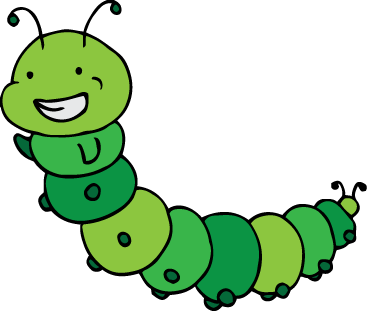The image features a digitally created, cartoonish caterpillar-worm against a white background. The caterpillar consists of ten round body segments in varying shades of green, ranging from light to dark and olive green. Its head is positioned at the top left, angling down towards the bottom right, suggesting a playful, rising motion. The caterpillar sports a cheerful expression with a big smile showing teeth, two small black eyes, and two black antennae protruding from the top of its head. Each body segment has little dark green feet, appearing as tiny circles, and the end segment also has a pair of small antennae. This whimsical creature appears to be in mid-wave, adding to its friendly and animated demeanor.